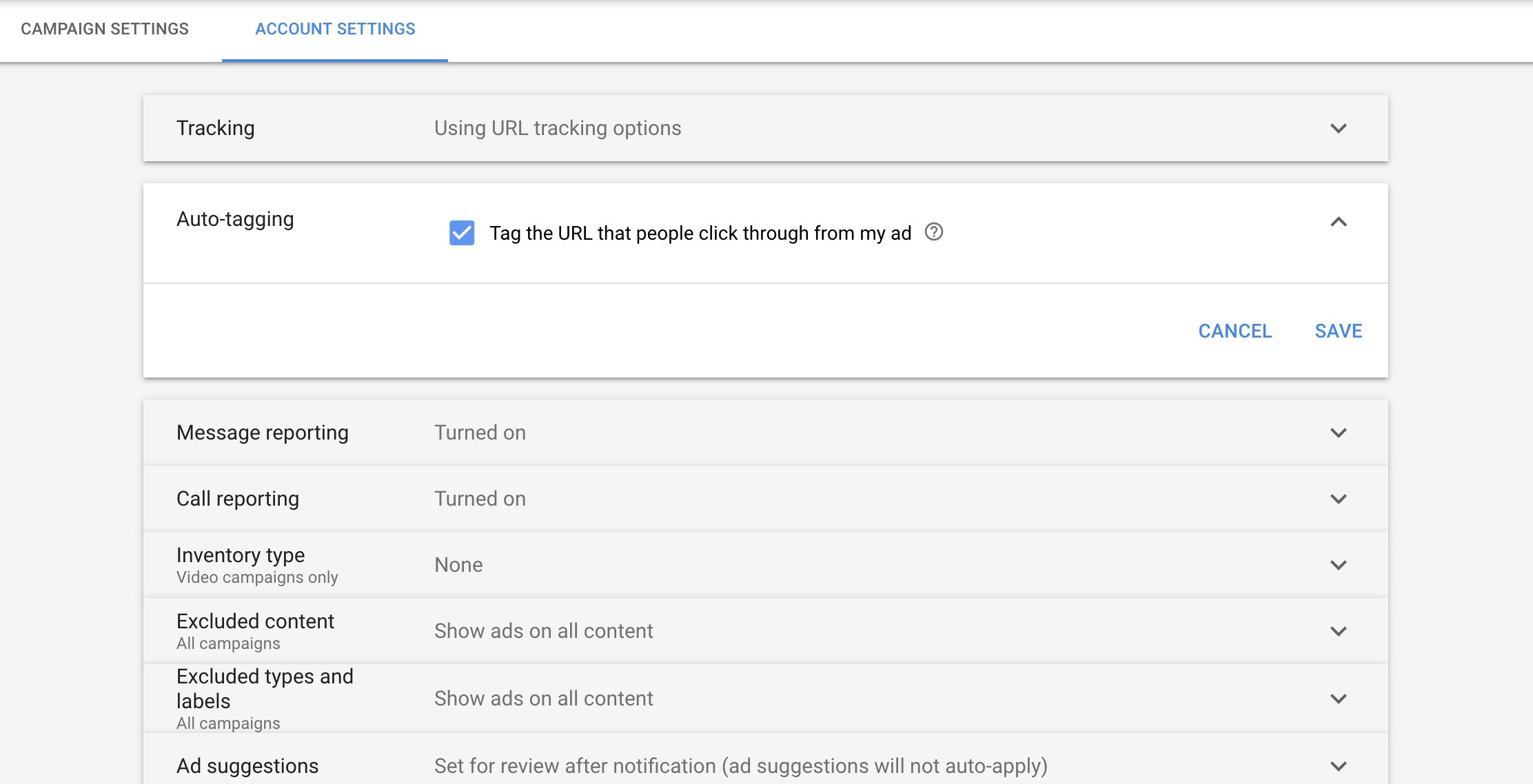The image is a screenshot from a website showcasing the "Campaign Settings" section. The layout begins with a white banner at the top, where "CAMPAIGN SETTINGS" is prominently displayed in black capital letters on the top left, and "Account Settings" is shown in blue, underlined text on the top right.

Below the banner, the background shifts to a light gray, featuring a large rectangle labeled "Tracking" with a capital T. This is followed by the section "Using URL Tracking Options," where "URL" is fully capitalized, indicating its importance. A drop-down menu is present beneath it.

Further down, another white banner appears, introducing the "Auto-Tagging" option with a capital A. A blue square with a white checkmark inside it is shown next to the text "Tag the URL that people click through my app," accompanied by an upward arrow. Below this, options to "Cancel" and "Save" are displayed in blue text.

The lower section of the image returns to a gray background. It lists several settings in a two-line format:

1. "Message Reporting: Turned On"
2. "Call Reporting: Turned Off"
3. "Inventory Type: Video Campaigns Only"
4. "Excluded Content: All Campaigns, Show Ads on All Content"
5. "Excluded Types and Labels: All Campaigns, Show Ads on All Content"
6. "Add Suggestions: Set for Review After Notification (Add Suggestions Will Not Auto-Apply)"

Each setting is accompanied by a drop-down menu, allowing for additional customization. The clear separation of sections and consistent use of color and capitalization enhances the readability and user experience.